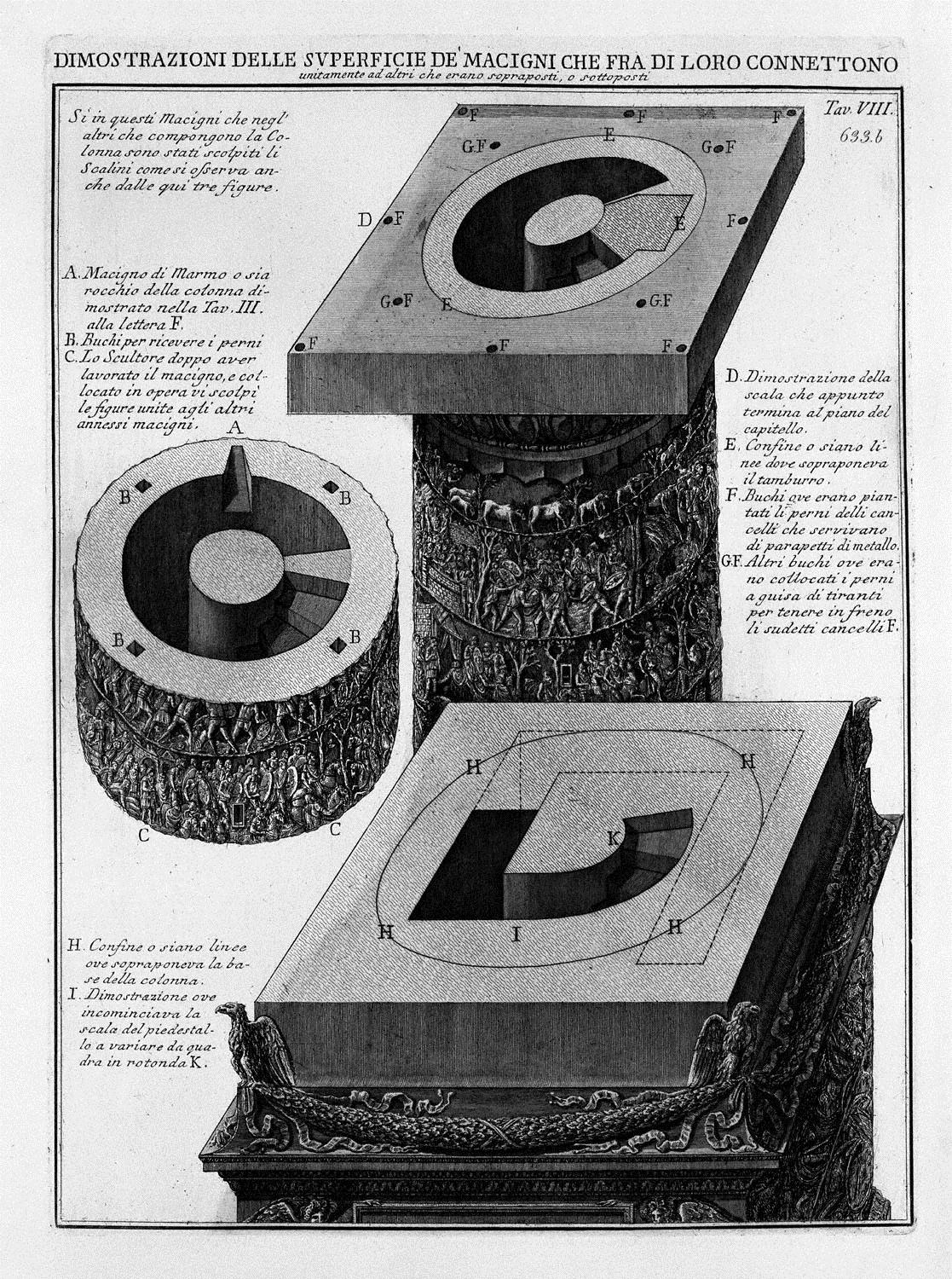This detailed black-and-white drawing appears to be an old patent illustration of a piece of machinery, complete with Italian text that seems to title it "dimonstrazioni del superficie del macchini cal freccia dell'oraconetto." The central elements in the foreground include a book resting on a table flanked by intricately detailed components. To the left, there's a cylindrical device marked with the letter 'B' and resembling a gear. Above this, a rectangular slab sits on a pedestal featuring another circular component similar to the one on the cylinder. The background has a considerable amount of script in Italian, possibly dating back many years, giving it an antique feel. The script surrounds the objects and might be instructions or labels corresponding to parts of the machinery, with letters A through G identifying each part. The ornate handles of the blocks display detailed carvings of people, horses, and other animals, suggesting the machinery's use in an old-timey printing press or for woodblock printing. The entire composition is rich in detail, framed by both white and black borders, and portrays a sophisticated and likely important piece of equipment from the past.